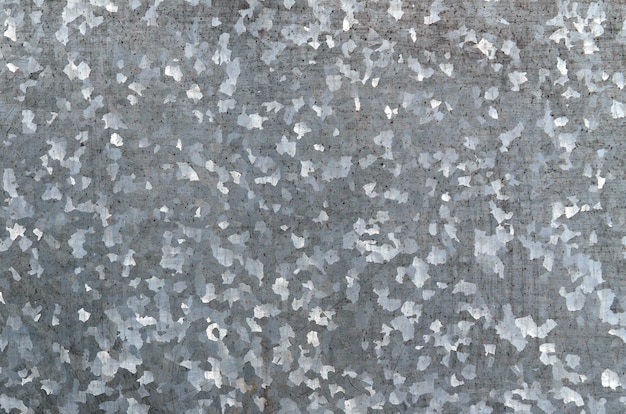The image features a rectangular composition, wider than it is tall, showcasing an abstract pattern that could be a painting or a close-up photograph of a textured surface. The backdrop is primarily grey, interspersed with various shades ranging from dark grey to almost black, with occasional hints of blue, and bright white spatters. The speckles are randomly distributed across the entire canvas, resembling tiny brush taps or flecks of splattered paint. Some spots appear more like smudges, adding to a pixelated and dappled effect. There's a sense of a metallic or rocky texture, suggesting the possibility of it being a photograph of a granite countertop or metal sheeting. The pattern lacks a discernible design, yet maintains a balanced and aesthetically pleasing monotone color scheme. Various-sized speckles, some as small as a quarter of an inch and others reaching up to an inch, along with sporadic darker blotches, contribute to the intriguing randomness of this visually textured image.